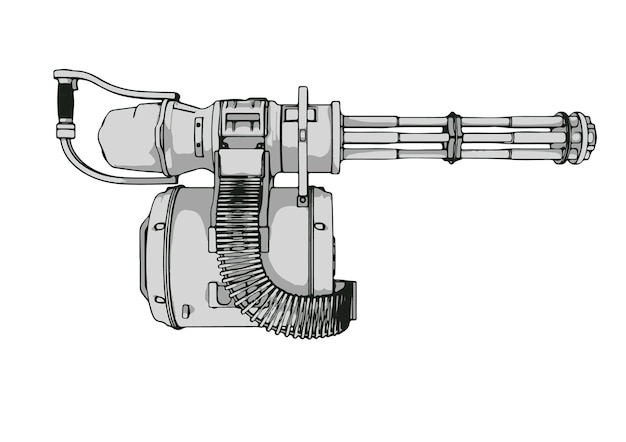This image depicts a detailed, drawn model of a rapid-fire military rifle or automatic weapon. The gun features three to four thin, multi-barrel extensions held together by steel plates at the top and middle of the device. Ammunition, arranged in a ladder-like formation resembling a strip of pins, is fed into the gun from the right-hand side, leading into a drum-like apparatus where the bullets are stored. A handgrip at the back provides stability for the shooter to handle the substantial kickback of the heavy machinery. The entire machine is rendered in light and medium gray tones, with distinguishing elements like the larger drum and a narrow cylinder, and a black handle at the rear contributing to the intricate design.